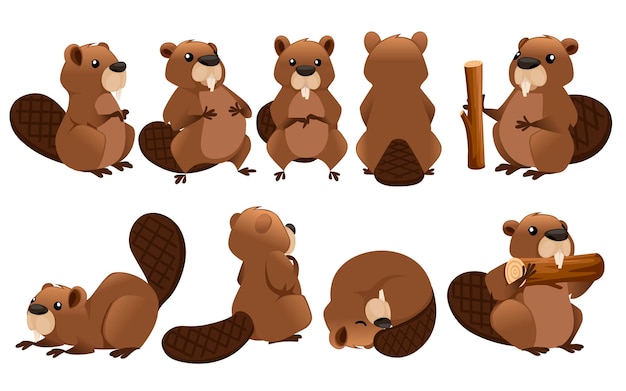The image is a collection of nine detailed vector illustrations of a cartoon beaver, showcasing various poses and angles for a character study. Positioned against a plain white background, these illustrations highlight the beaver’s playful and expressive nature. The beaver is primarily brown, with a very dark brown, crisscross-patterned tail, and has large eyes with white highlights for added detail and emotion. The sequence begins with the beaver in a side profile, facing left to right, followed by the beaver clutching its chest with both hands. Next, it is depicted facing forward with hands touching, then showing its back. Another illustration features the beaver holding a piece of wood. The bottom row includes the beaver on all fours, then from the back, curled up as if sleeping, and finally, joyfully gnawing on a piece of wood. Each pose brings out the beaver's endearing and excitable personality, making it a charming vector set ideal for various design projects.